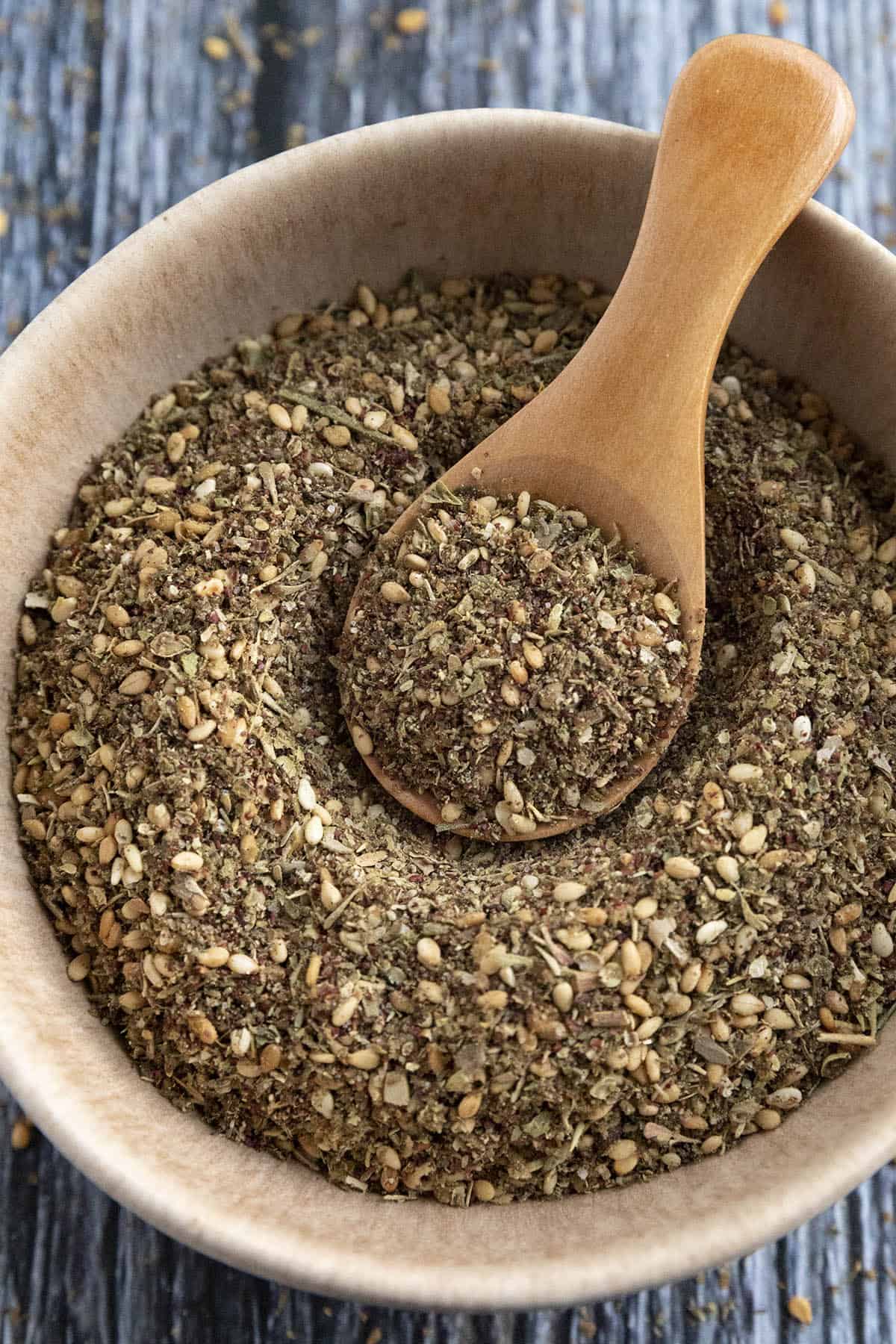This high-quality photograph, likely taken by a professional or an avid hobbyist, captures an overhead view of a rustic setting featuring a tan ceramic bowl filled with a mixture of ground-up herbs and various-sized seeds, including sesame seeds and possibly some olive green spices. Centered in the bowl is a small wooden spoon with a short handle, resting in an indentation it created when scooping the contents. The bowl, which has a dull and unfinished appearance, is set on a weathered, gray wooden tabletop. The wooden spoon, slightly darker than the bowl, leans against the bowl's lip, emphasizing the detailed textures and contrasts of the scene. The natural lighting enhances the earthy tones and the artisanal feel of the setup.